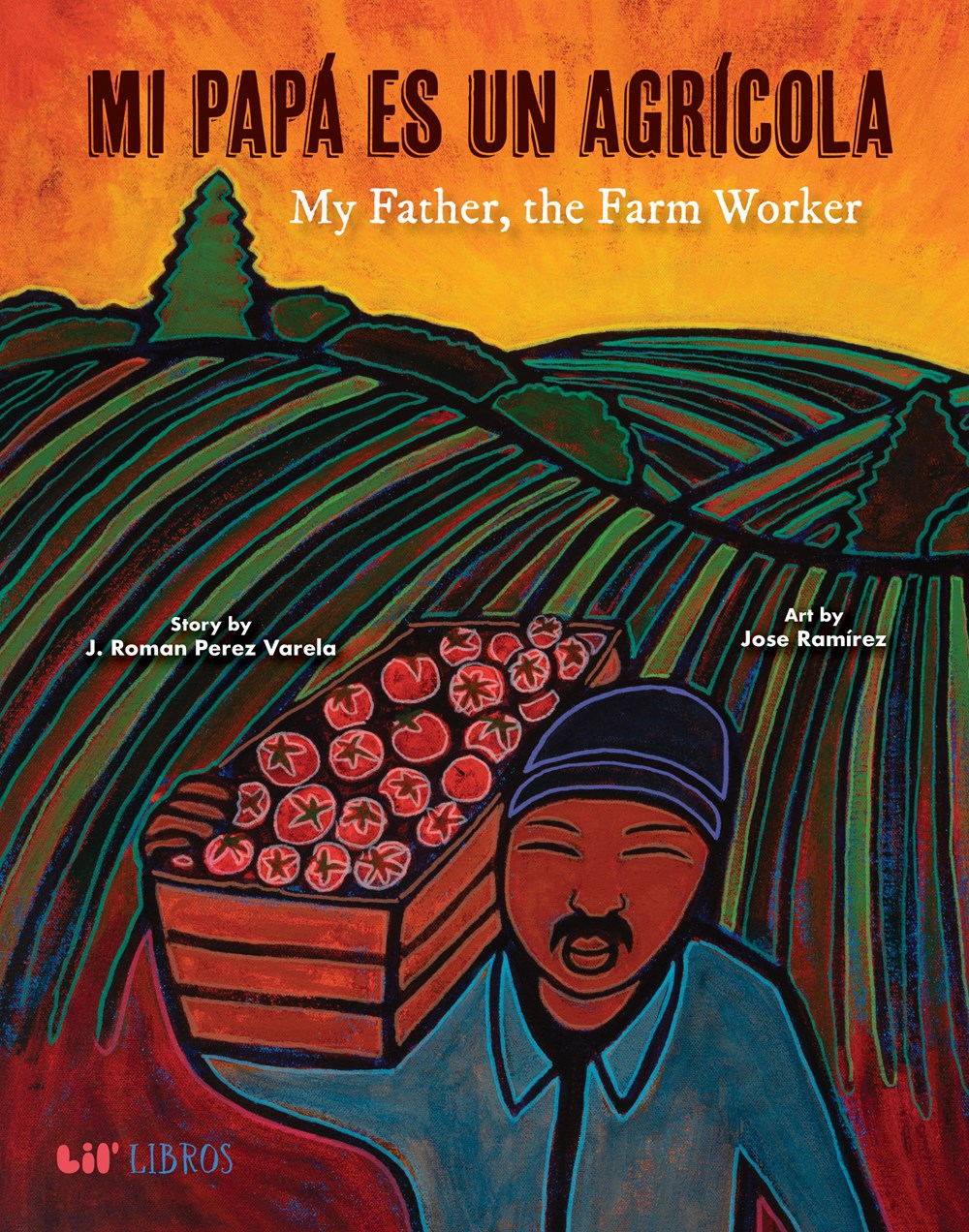The image is a vibrant and stylized book cover titled *Mi Papa es un Agricola*, with an English translation *My Father, the Farm Worker* written underneath in white. It features a colorful, painted landscape characterized by rolling hills in various shades of green, blue, black, and purple, set against a bright yellow-orange sunset sky. In the foreground stands a man with dark skin, wearing a bluish collared shirt and a hat, hoisting a large crate of tomatoes on his shoulder. The text in the middle of the cover credits the story to J. Roman Perez Varela on the left and the art to Jose Ramirez on the right. At the bottom of the image, the text reads "Little Libros." The overall effect is a richly colored and dynamic portrayal of agricultural life.